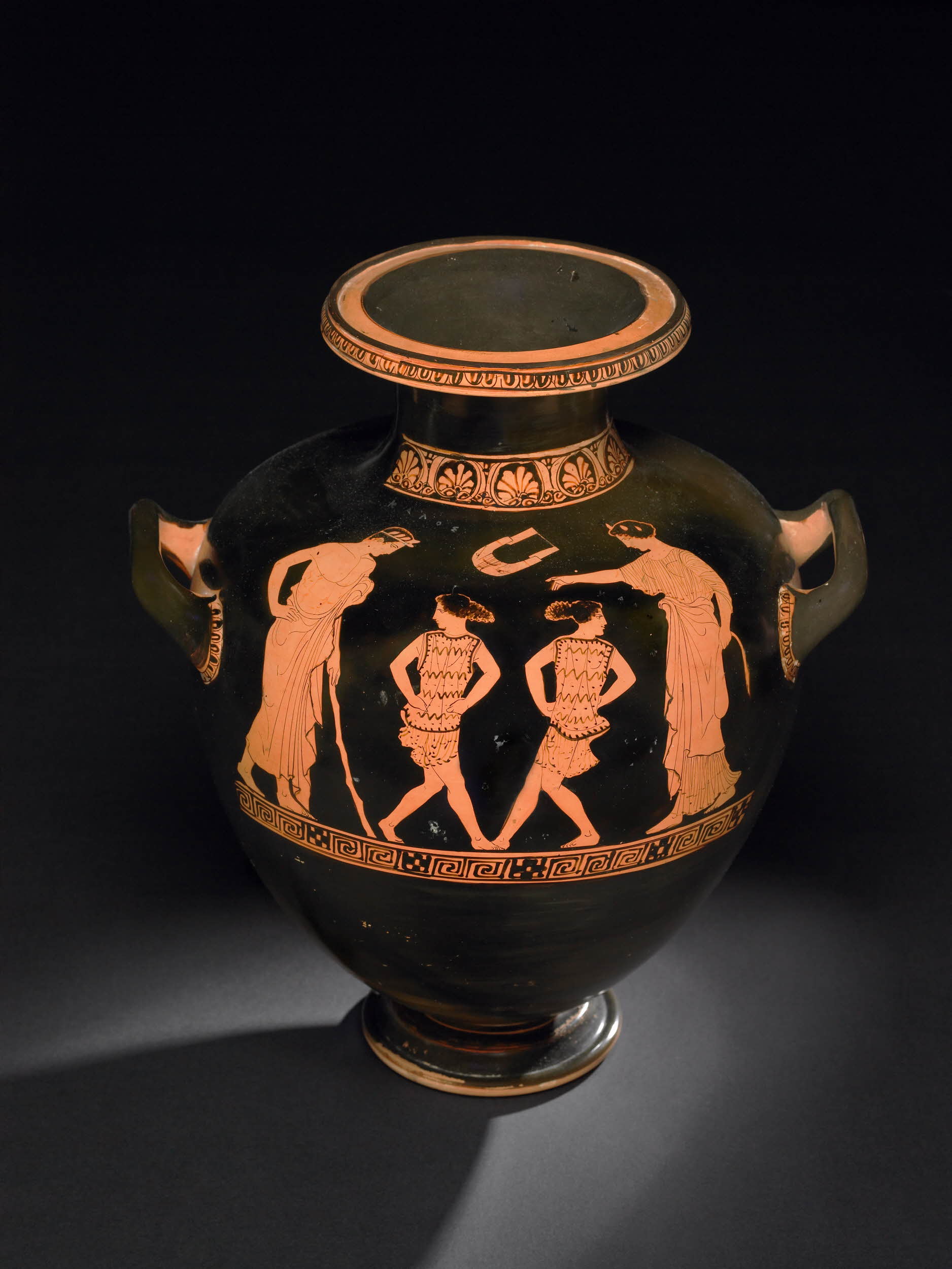This image captures a detailed black vase or urn, possibly of ancient Roman or Greek origin, hinting at a classical era. The vase features intricate designs in clay-colored etchings contrasted against its black background. These designs depict four figures: two central smaller figures, likely women, dressed in patterned frocks with one knee bent, touching toes, hands on their hips, and heads turned outwards. Flanking them are two larger figures dressed in togas. On one side, a man holding a cane appears to be pointing, while on the opposite side, another man looks downward, possibly in contemplation. Above the central figures, a floating harp-like instrument is intricately etched, adding to the scene’s dynamic feel. Ornamental tribal borders decorate the vase's lid, neck, and midpoint. Distinctive yellow highlights trim the figures and adorn the circular top, while the vase's substantial form is complemented by two prominent handles on either side.